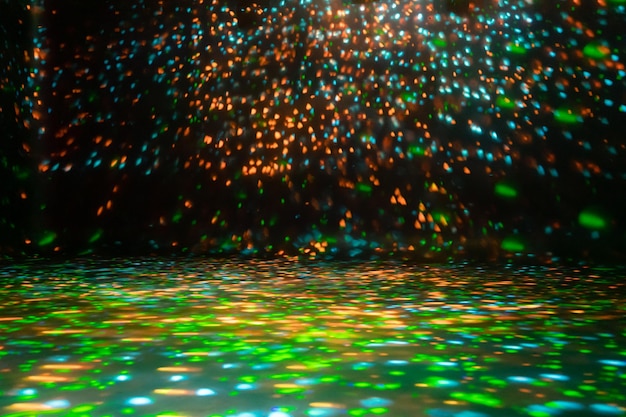The image presents a scene evocative of a 1970s roller disco or a dance floor, dominated by vibrant yellow, blue, green, and occasional red lights. These lights radiate from a central, undisclosed light source, assumed to be a disco ball or similar device situated above the frame. The lights create a mesmerizing, circular pattern that spills vividly across both the floor and the walls, enhancing the abstract and colorful composition of the scene. The interplay of these lights, reminiscent of a Monet painting, transforms the floor into a tapestry of bright green, blue, and orange patches, while the wall—curving gently upwards—captures sharper, more distinct points of red, blue, and green. The dark, almost indiscernible walls serve as a canvas, amplifying the visual effect of the lights, making it appear as though the entire scene is within an expansive, dimly lit room solely illuminated by this dynamic light display. No other objects or people are present in the photograph, heightening the focus on this ethereal spectacle of light.